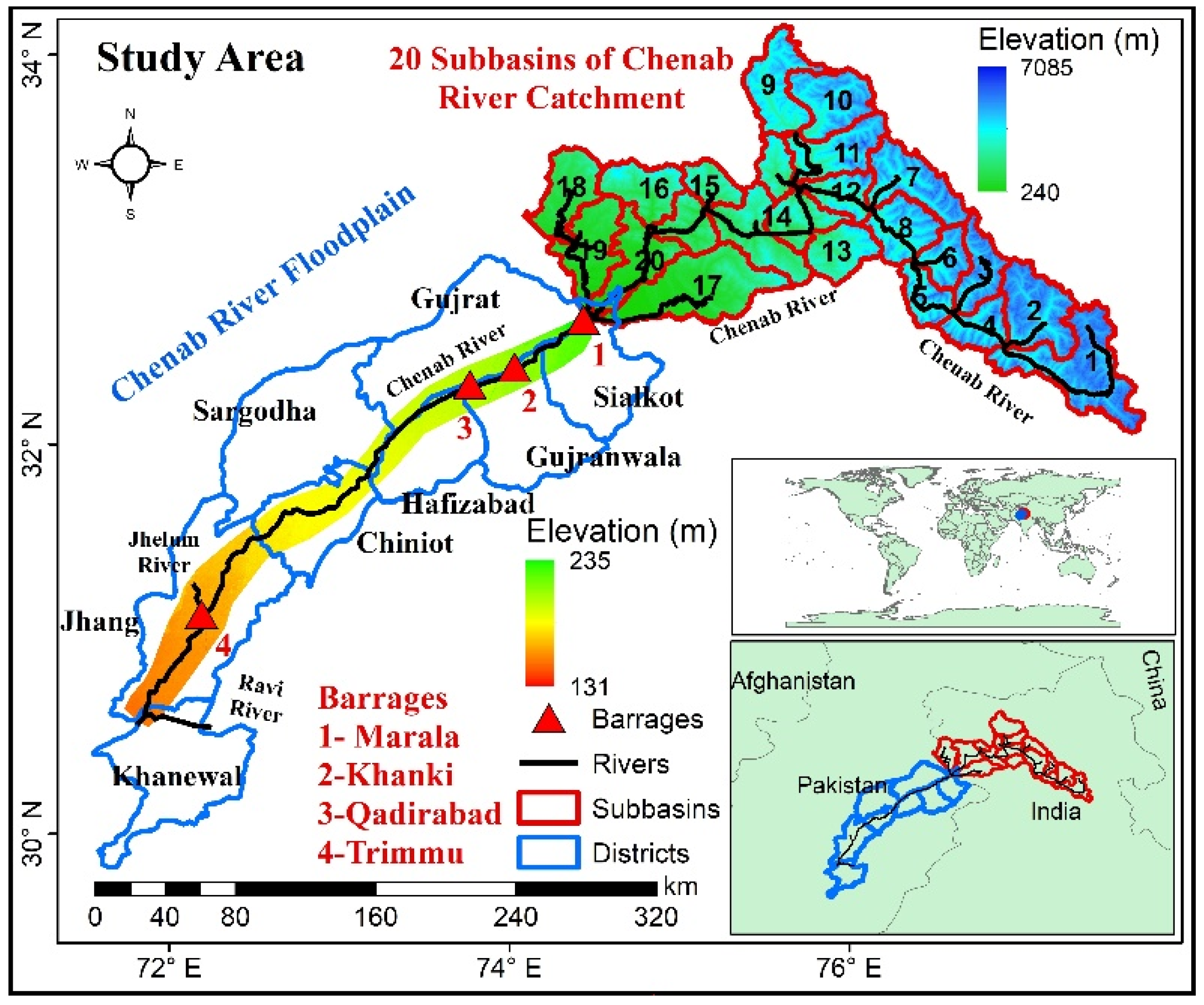This detailed map depicts the Chenab River floodplain, covering regions of Afghanistan, Pakistan, India, and China. The map is set against a white background with black writing and includes a coordinate grid marking degrees around its perimeter. Detailed topographic elements are represented with an elevation chart, featuring a color scheme where low elevations are indicated in red, medium elevations blend from green, and high elevations are in blue. Key features like rivers, barrages, sub-basins, and districts are highlighted with specific symbols: red triangles for barrages, black lines for rivers, red rectangles for sub-basins, and blue rectangles for districts. The map lists notable barrages such as Maralla, Kanki, Khwadirabad, and Trimu. Additional inset maps at the bottom provide context with smaller-scale detail, including a global location map. Black lines and labels indicate major rivers and reference numbers give geographic coordinates, allowing a comprehensive understanding of the elevation and geographic elements of the study area.